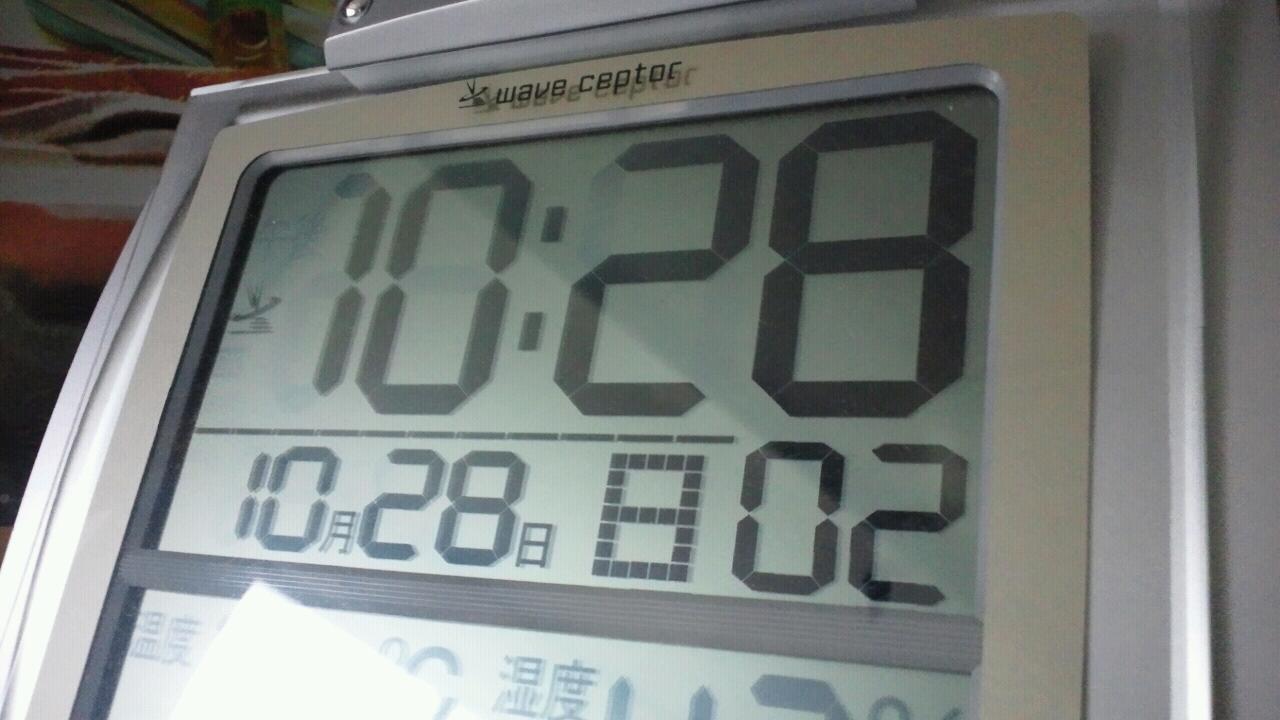This is a close-up, horizontal, color photograph of a digital clock or potentially a weather station device. The device has a rectangular, gray, silver-toned casing. At the top of the LCD display, the brand name "Waveceptor" is clearly visible, written in black lettering. The display shows the time "10:28" prominently in bold numbers. Beneath the time, the date is displayed with "10" followed by either Japanese or Chinese characters for month and day, and then the number "28." There's an additional pixelated "8" and the number "02," representing seconds, also visible. The lower portion of the display includes symbols indicating temperature (in degrees Celsius) and humidity level. The upper left corner of the image features a slight orangey background tint. The overall photograph centers the device, but the bright light obscures some of the bottom details of the display, emphasizing the primary time and date information.